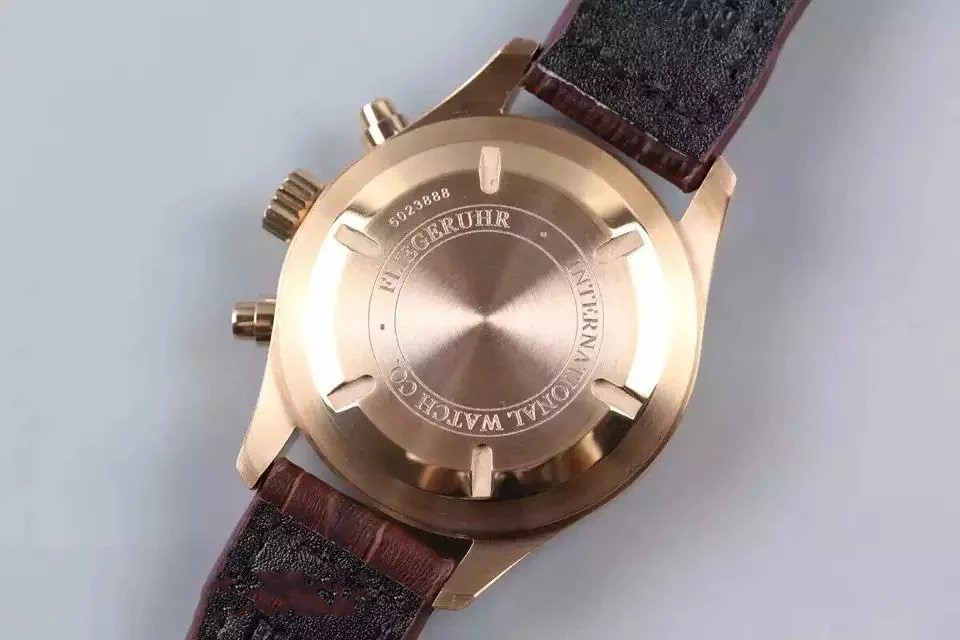This close-up photograph showcases the intricate design on the back of a wristwatch. The focal point of the image is a circular medallion made of light brown metal, elegantly placed at the center. Encircling this medallion is a double-ring engraving, within which delicate writing is inscribed, adding a touch of sophistication. Emanating from the central circle, finely etched lines radiate outward, reminiscent of sun rays. Positioned to the left center is the watch's winding knob, a striking gold-bronze color that stands out. Flanking the knob are two cone-shaped accents that extend to either side. The watch band, visible at the edges, features a rich brown exterior, while the underside is contrasted in black, showcasing a seamless blend of materials and craftsmanship.